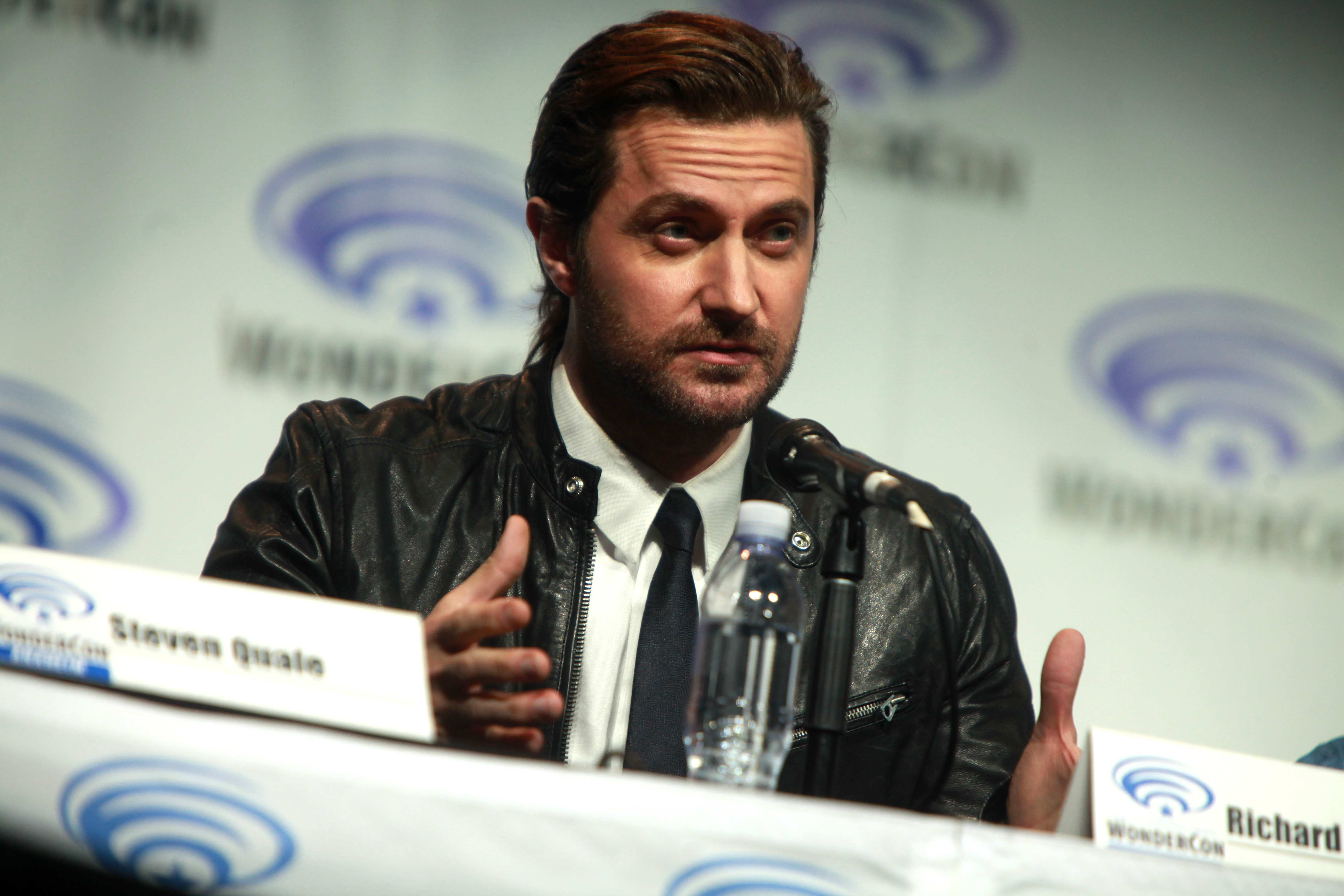The image depicts a serious-looking man with reddish brown hair and a beard, sitting at a press conference panel at WonderCon. He is captured mid-speech, gesticulating with both hands while seated in front of a table that has a reflective, light blue surface with a swirly logo. The professional photograph appears to have been taken from a low angle, and a white banner with a blue logo and black text forms the backdrop. The man is dressed in a white button-down shirt, a black or navy tie, and a black leather jacket. In front of him is a bottle of water and a name card that reads "Richard." To his right is another name card labeled "Stephen Quayle." The image's colors include black, white, gray, brown, peach, and various shades of blue, enhancing the formal and professional atmosphere of the event.